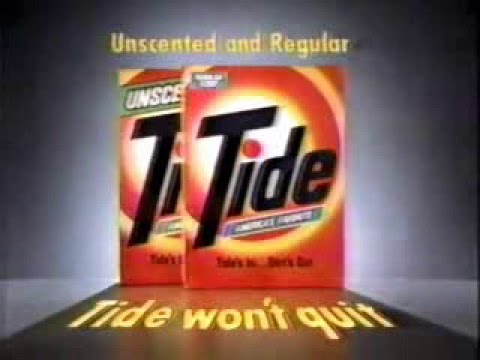The image is an old-fashioned, retro-style advertisement for Tide detergent, featuring two orange-colored boxes with bold black lettering spelling "Tide." The "i" in "Tide" is accented with a red dot, and the boxes are adorned with yellow and orange around the letters. The two boxes, which are square-shaped and contain powder detergent, are placed side by side, slightly overlapping, with a green label indicating the product as "unscented." At the top of the image, in yellow font, the words "unscented" and "regular" are clearly visible, while below the boxes, the text "Tide Won't Quit" is prominently displayed. The overall image has a faded, blurred look with a gray background, giving it a distinctive antique or vintage feel, enhanced by shadows and a central light that fades off into darkness at the edges.